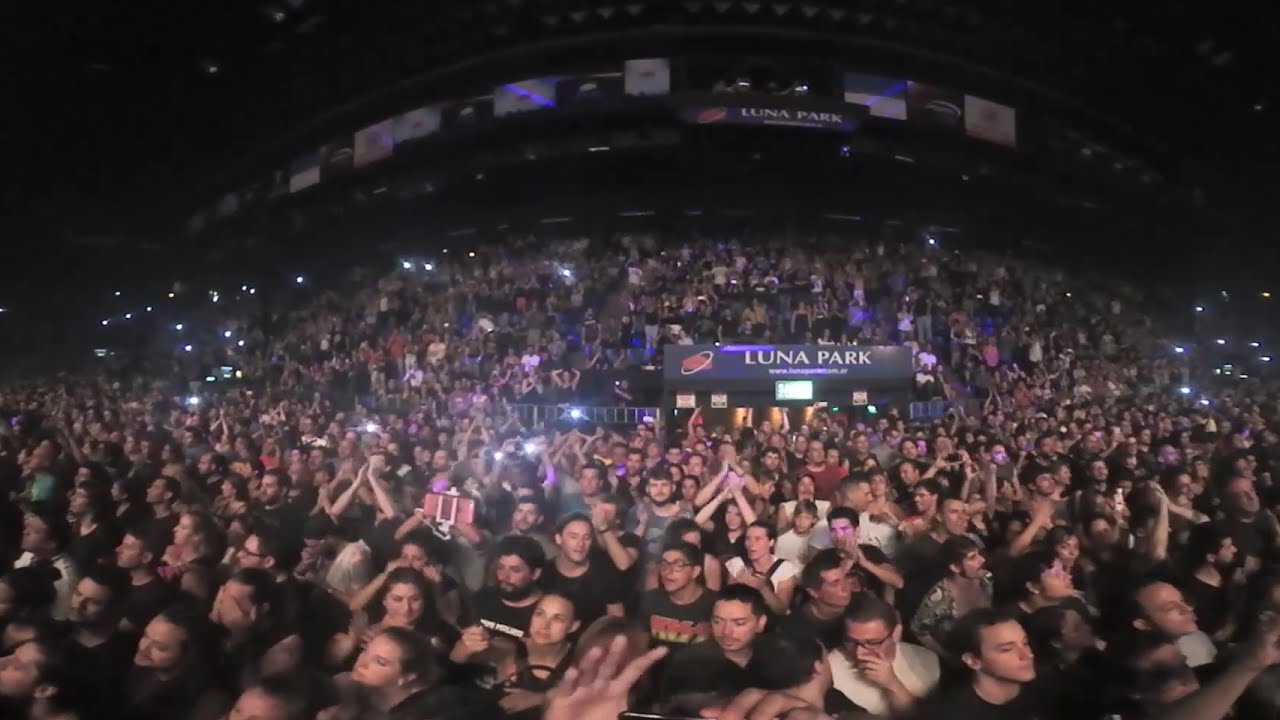The image captures a densely packed crowd at an outdoor concert at Luna Park, evident from multiple black signs bearing the name "Luna Park" and an illustration of a red planet with a white ring. Toward the middle right and top of the image, these signs are prominently displayed. The upper portion of the image is dominated by a dark background with various hanging signs, some of which are white, and several lights illuminating the scene. The crowd, filling the middle to the bottom of the image, is vibrant and lively, with people clapping, waving, and talking to each other. Some fans are using their cell phones to create lights. The stadium seating rises at an angle from the standing area, indicating a large, multi-level venue. Notable is a spectator wearing a KISS t-shirt, adding to the concert atmosphere. Above the crowd, jumbo screens broadcast indistinct images, surrounded by advertisements hanging in the rafters.